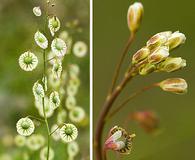The image is a very small, side-by-side composition of two portrait-style photographs with a thin white line separating them. On the left, the photo features a plant with a slender green stem branching out into multiple smaller stems, each capped by green balls encircled by white rings, reminiscent of magnified tiny buds or possibly dandelions. The background is blurred, showing indistinct green foliage that adds depth to the scene. On the right, the second photo presents a different plant with a more woody, brown stem that curves upward, adorned with numerous buds. These cream-colored buds have hints of reddish, dark red, or brown tones. One bud at the bottom is partially open, revealing more vibrant red and white hues. A colorful, heart-shaped leaf with white, pink, and orange patches grows lower on the stem, adding to the intricate details of the composition. The background here is also blurred, with vague shapes of additional flowers contributing to the overall verdant ambiance.